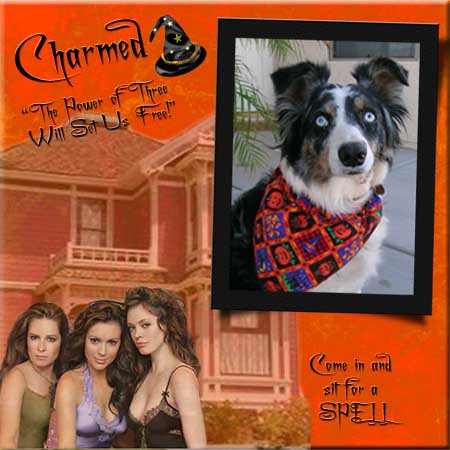This Halloween-themed promotional graphic for the television show "Charmed" features an orange background and a blend of mystical and seasonal elements. In the top left corner, the iconic "Charmed" logo is paired with a small, black witch's hat. A quote from the show, "The power of three will set us free," is displayed prominently. The upper right section showcases a black-and-white dog with striking blue eyes, adorned in a festive red and pumpkin-themed bandana, adding a cute and spooky touch. The bottom left corner highlights an image of the three main actresses from the show, each dressed in green, purple, and black tops. They all have long wavy brown hair and stand in front of the Charmed house, which is subtly visible in the background. A final touch, "Come in and sit for a spell," invites viewers into the enchanting world of Charmed.